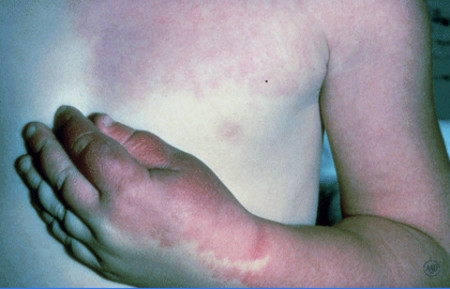The image captures the left pectoral area, shoulder, and full length of the left arm of a young Caucasian male, revealing a pronounced and unusual rash. The affliction starts above his left nipple, spanning across the chest to the armpit, and continues over the shoulder down to the wrist. Remarkably, the thumb, index, and middle finger are also affected, appearing swollen and intensely red, while the rest of the hand remains unaffected. The rash has distinct jagged edges and contrasts sharply with the surrounding normal white skin, emphasizing its severity and irritation. In the background, visible only in small patches, there are hints of blue and black below his armpit and in the upper right corner, though the primary focus is on the inflamed and swollen areas of his skin.